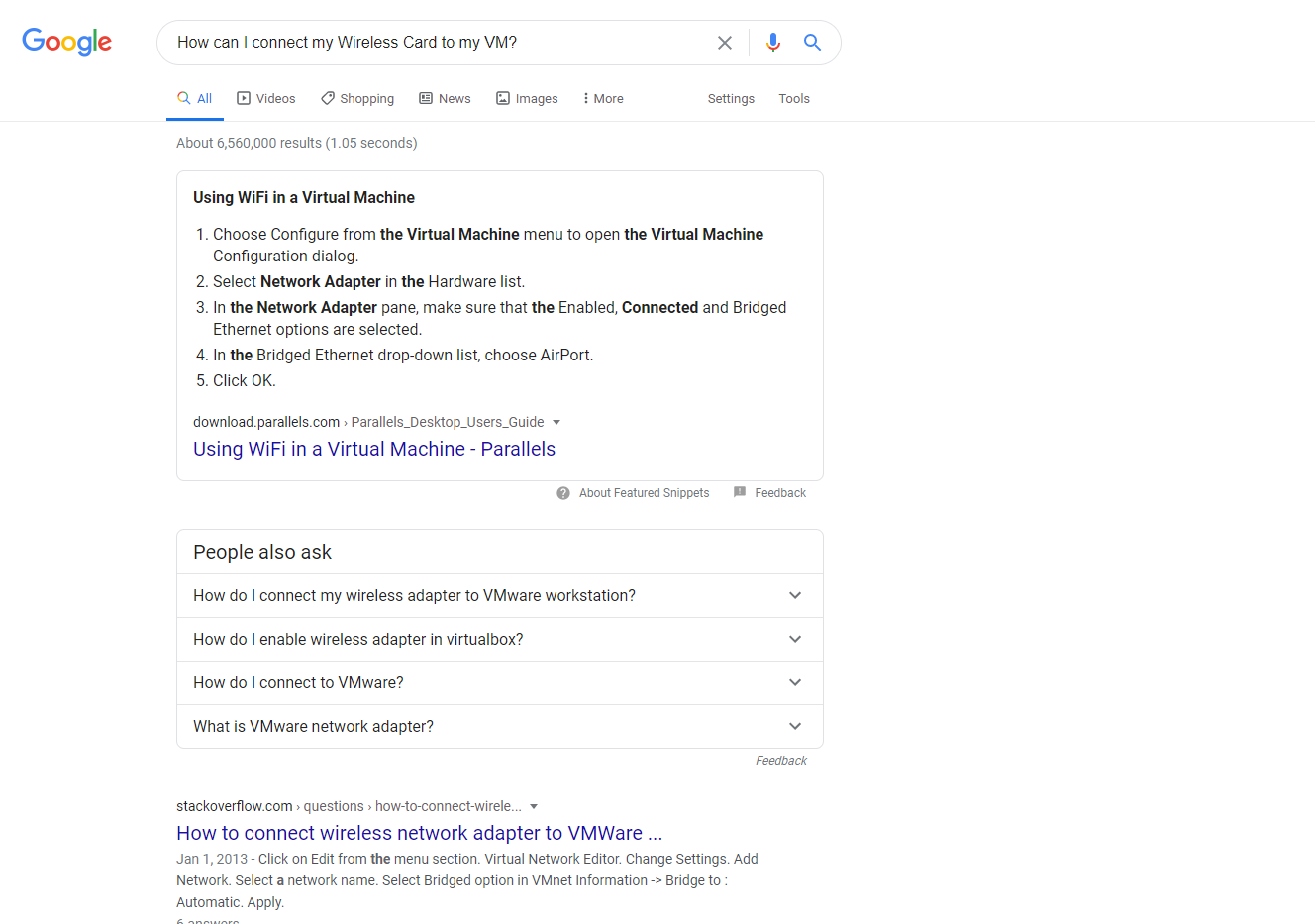A screenshot of a Google search results page with various elements related to the query, "How can I connect my wireless card to my VM?" is prominently displayed. At the top left, the multicolored Google logo is visible, and the search bar contains the aforementioned query, ending with a question mark.

Just below the search bar, the familiar tabs for "All," "Videos," "Shopping," "News," "Images," and "More" can be seen, with "All" being underlined, indicating it is the selected tab. Approximately 6,560,000 results have been found in 1.05 seconds.

The first result is highlighted in a gray outlined box titled "Using Wi-Fi in a Virtual Machine" from downloadparables.com. It provides a step-by-step guide:
1. Choose "Configure" from the virtual machine menu to open the configuration dialog.
2. Select "Network Adapter" in the hardware list.
3. Ensure the "Enabled," "Connected," and "Bridged Ethernet" options are selected in the network adapter pane, and choose "Airport" from the bridged Ethernet drop-down list.
4. Click "OK."
The source is cited as downloadparables.com, specifically from a Parallels Desktop user guide.

Below this, there is information about featured snippets and feedback.

The next gray outlined box lists "People also ask" with expandable questions:
- How do I connect my wireless adapter to VMware Workstation?
- How do I enable wireless adapter in VirtualBox?
- How do I connect to VMware?
- What is VMware network adapter?

Following this is a feedback option.

Further down, the second result, from stackoverflow.com, is partially visible with a truncated title, "How to connect wireless network adapter to VMware..." dated January 1, 2013. It suggests editing from the menu selection, accessing the virtual network editor, changing settings, adding a network, naming the network, selecting the bridge option in VMnet information, and applying the changes.